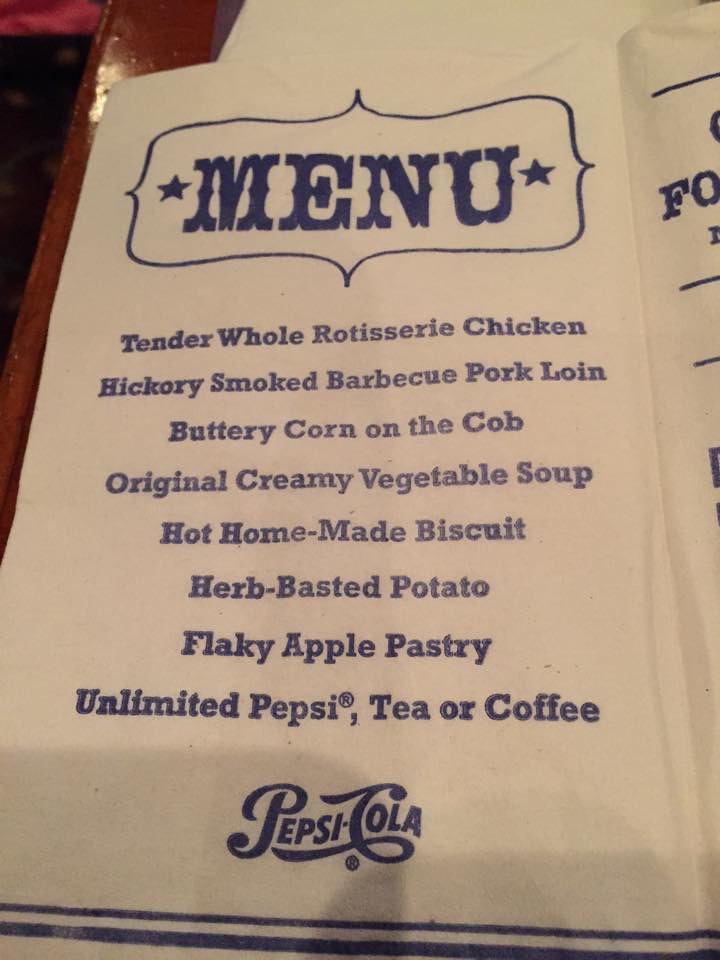The image captures an up-close, slightly angled view of a menu resting on a brown table. A pink object can be seen in the background, adding a pop of color to the scene. The white piece of paper underneath the menu is partially visible, accentuated by the menu's noticeable creases—both at the top and extending towards the bottom. Shadows are cast on the bottom part of the menu, possibly reflecting the photographer's cell phone.

The menu itself features the word "MENU" in uppercase blue letters, encased in a decorative box with stars on either side. The food choices listed include:
- Tender whole rotisserie chicken,
- Hickory smoked barbecue pork loin,
- Buttery corn on the cob,
- Original creamy vegetable soup,
- Hot homemade biscuit,
- Herb basted potato,
- Flaky apple pastry.

At the bottom, the menu highlights "unlimited Pepsi, tea, or coffee" and prominently features the "Pepsi Cola" logo in a distinctive font. The final portion of the page is not fully visible, showing only some lines and words in blue.